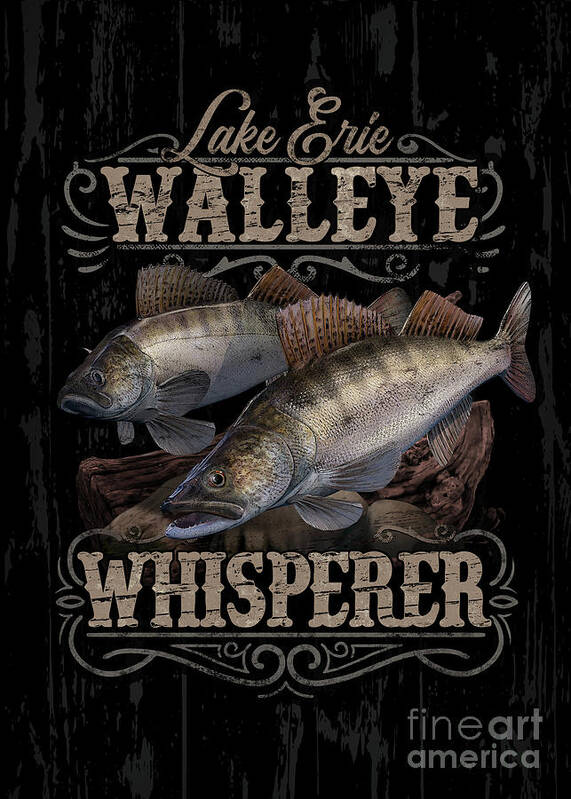This digitally rendered poster features a striking composition centered on two Lake Erie Walleye fish, depicted with meticulous detail. These fish are rendered with spined fins at the tops of their bodies and distinct stripes running halfway down their sides. One fish has its mouth open, while the other has its mouth closed, with one positioned slightly in front of the other, partially obscuring the fish in the background. They are oriented to the left, showcasing a gradient coloration from greenish on the top ridge fading to silver beneath.

The backdrop of the image is a sophisticated black with a subtle gray wood grain texture, simulating the appearance of aged wood paneling. Enhancing its vintage aesthetic, the poster is adorned with ornate gold lettering in an Old Western style font. At the top, it proclaims "Lake Erie Walleye Whisperer," indicative of a specialized, perhaps local, connection to fishing for this specific species. Below these elements, and complementing the design, is the watermark "Fine Art America" in matching gray lettering, anchoring the bottom right corner and attributing the artwork. This piece cleverly combines a classic, rustic charm with digital precision, appealing to fishing enthusiasts and art collectors alike.